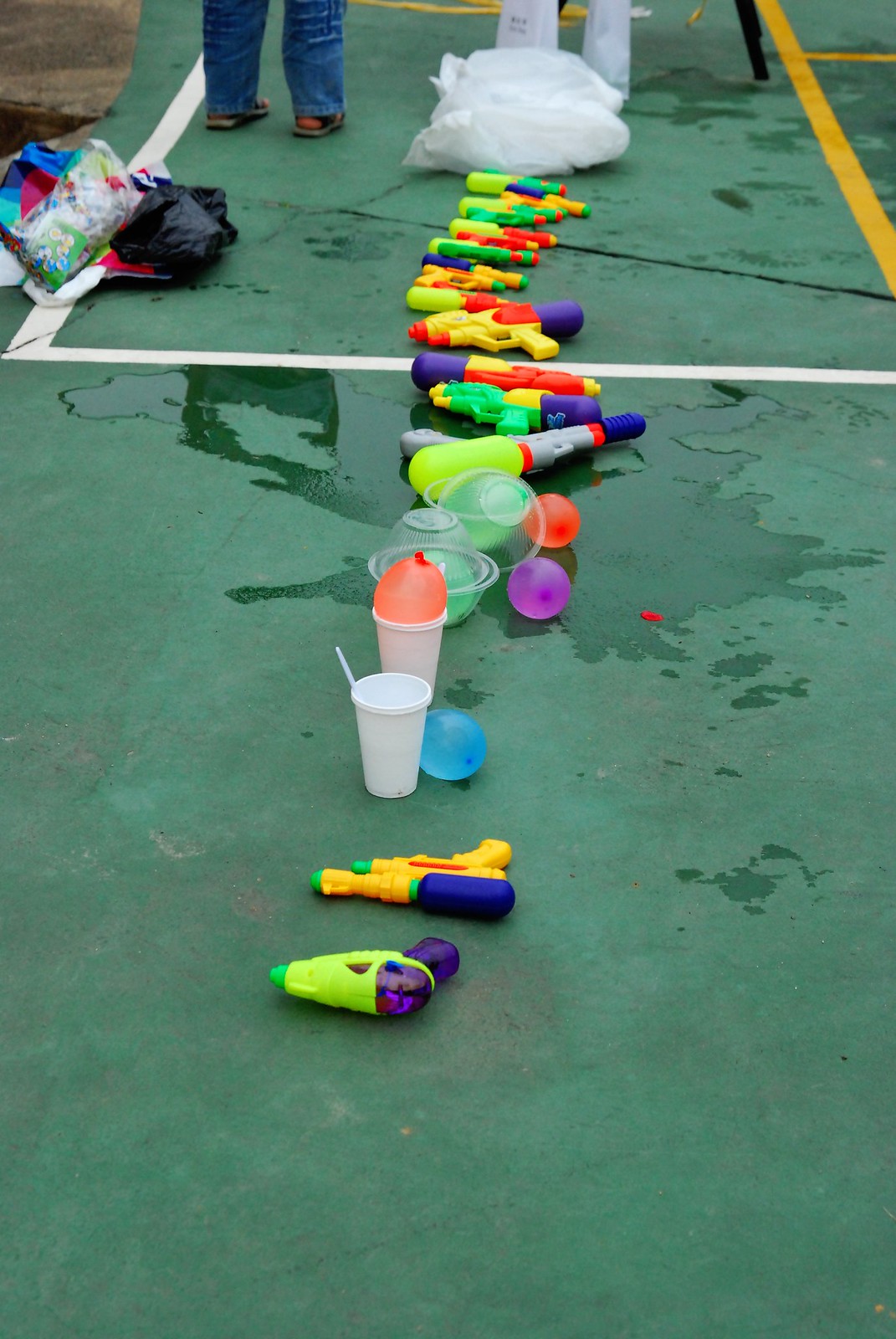The photograph, taken during an overcast day, captures a green-painted court, possibly for tennis or pickleball, with both white and yellow boundary lines. Dominating the center of the image, there is a neat lineup of brightly colored water guns in various shapes and sizes, featuring hues of green, yellow, red, and purple. Beneath the water guns, a small puddle has formed due to the leaking water. Scattered among the water guns are water balloons, Styrofoam cups, and some light green plastic bowls. In the background, the lower legs of people are visible; one individual to the right is wearing blue jeans and sandals. Piled up in the back are white plastic bags and additional bags that appear to contain more water balloons. The ground is wet, indicating recent water activity, enhancing the playful and vibrant scene depicted.